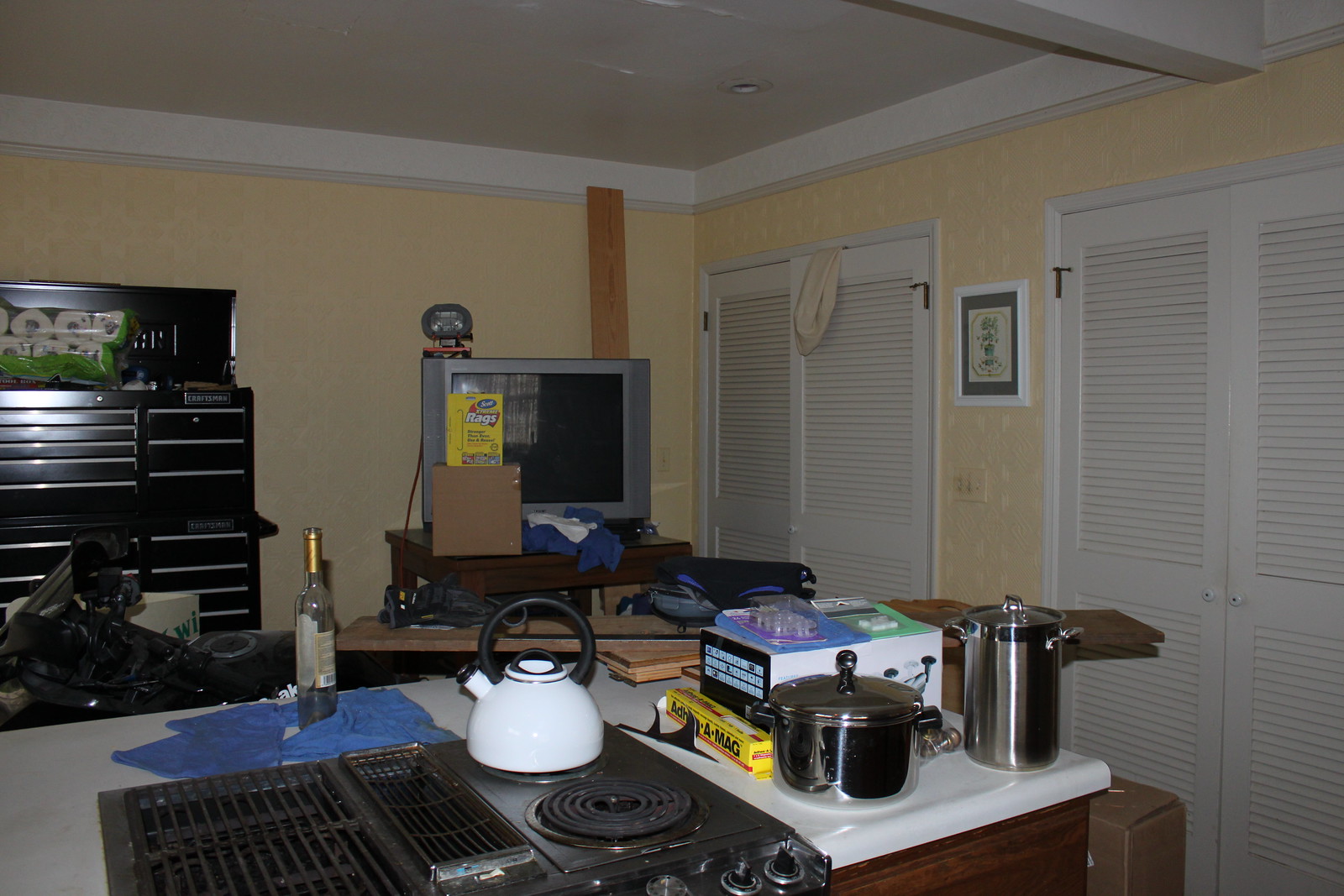The photograph captures a seamless blend of a kitchen and living room within a home. This rectangular image shows the top and bottom sides elongated compared to the left and right sides. The walls of the room are adorned with yellow wallpaper, accented with slightly lighter yellow dots, imparting a sunny and inviting atmosphere. On the right side, there's a double-door closet with slatted panels, each door equipped with small, round white knobs and brass-colored hinges. An identical set of doors is located on the opposite end of the room, providing symmetry.

Between these doors, a framed piece of artwork featuring a plant set on a white background with a gray border adds a touch of elegance. The frame is simple yet sophisticated in white. The ceiling is painted white, and features round recesses that likely house lights for subtle illumination. A prominent long white support beam spans the ceiling's upper right corner, enhancing the room's structural aesthetic.

In the kitchen area, located in the bottom left of the image, a stylish kitchen island counter stands out with its pristine white countertop. Centrally positioned on the island is a black cooktop; the left half functions as a grill, while the right half includes two round burners. Resting on the back burner is a white tea kettle with a round black handle, ready for use. The image overall exudes a warm and cozy ambiance while maintaining a modern, functional living space.